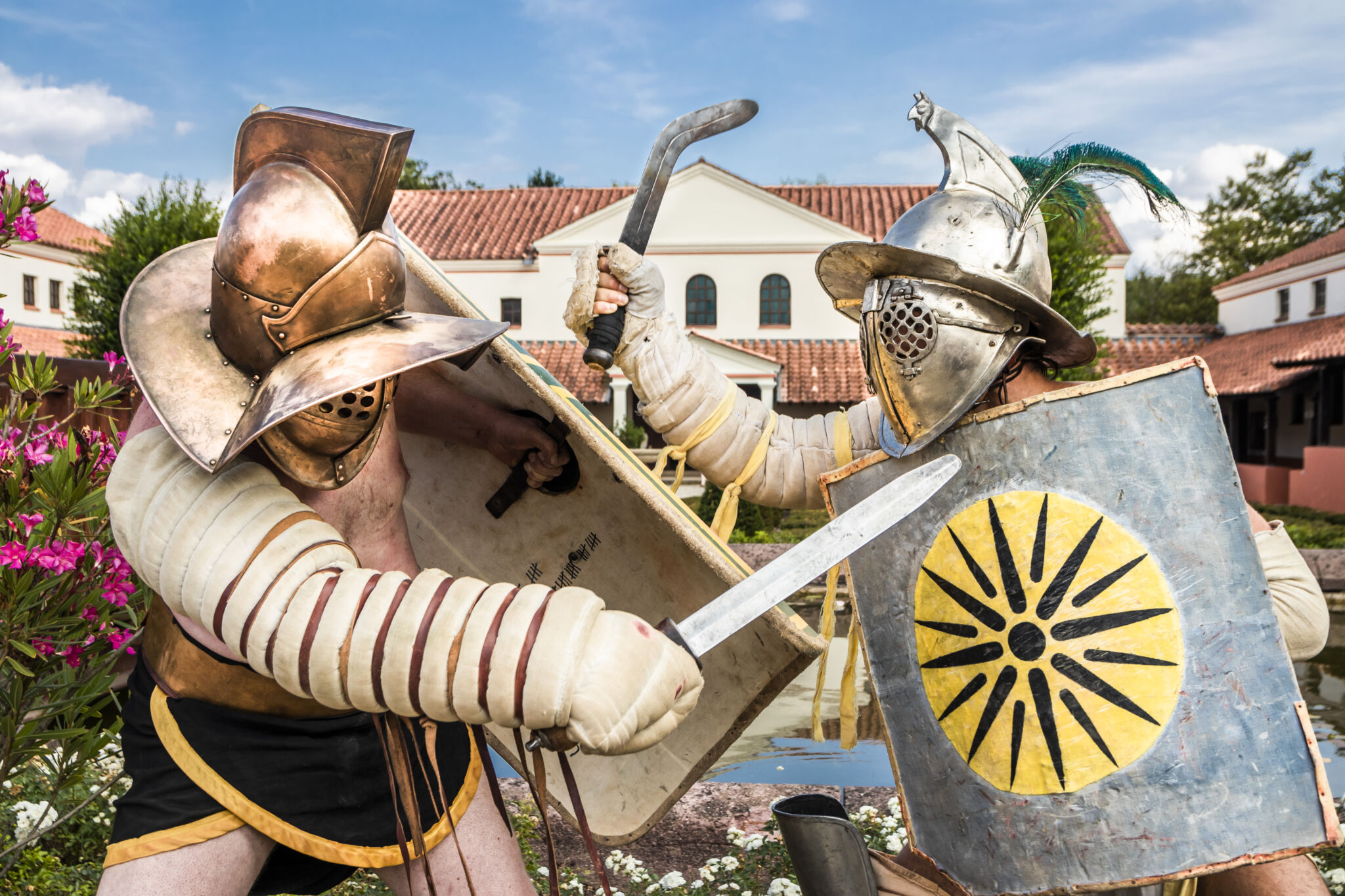The daytime outdoor photograph captures a strikingly detailed scene set in the courtyard of a villa. In the background, a whitewashed building with a brown tile roof stands against the mostly blue sky, punctuated by wispy white clouds. The courtyard is bordered by lush greenery and water features, enhancing the historical ambiance.

In the forefront, two men are engaged in a fierce gladiatorial battle. Both warriors are clad in elaborate, ancient-style armor made of metal, with distinct differences in their gear's appearance and coloration. Their heavy helmets are designed with narrow eye slits and a protective brim, obscuring their faces but allowing for a sense of intensity and mystery to the scene.

The man on the left wears a copper-colored helmet and black skirt adorned with a golden border. His right arm is wrapped in a thick, cushioning fabric, and he brandishes a short sword while holding a large shield. His opponent on the right is dressed in a more chrome-toned armor. Similar fabric protection covers his right arm, and he wields a unique curved knife. His large shield features a formidable sunburst design, with a dark border and a central yellow circle radiating black rays.

Both men are mid-strike, their weapons clashing as they battle under the open sky, creating a dynamic and vivid depiction of this ancient combat scenario.